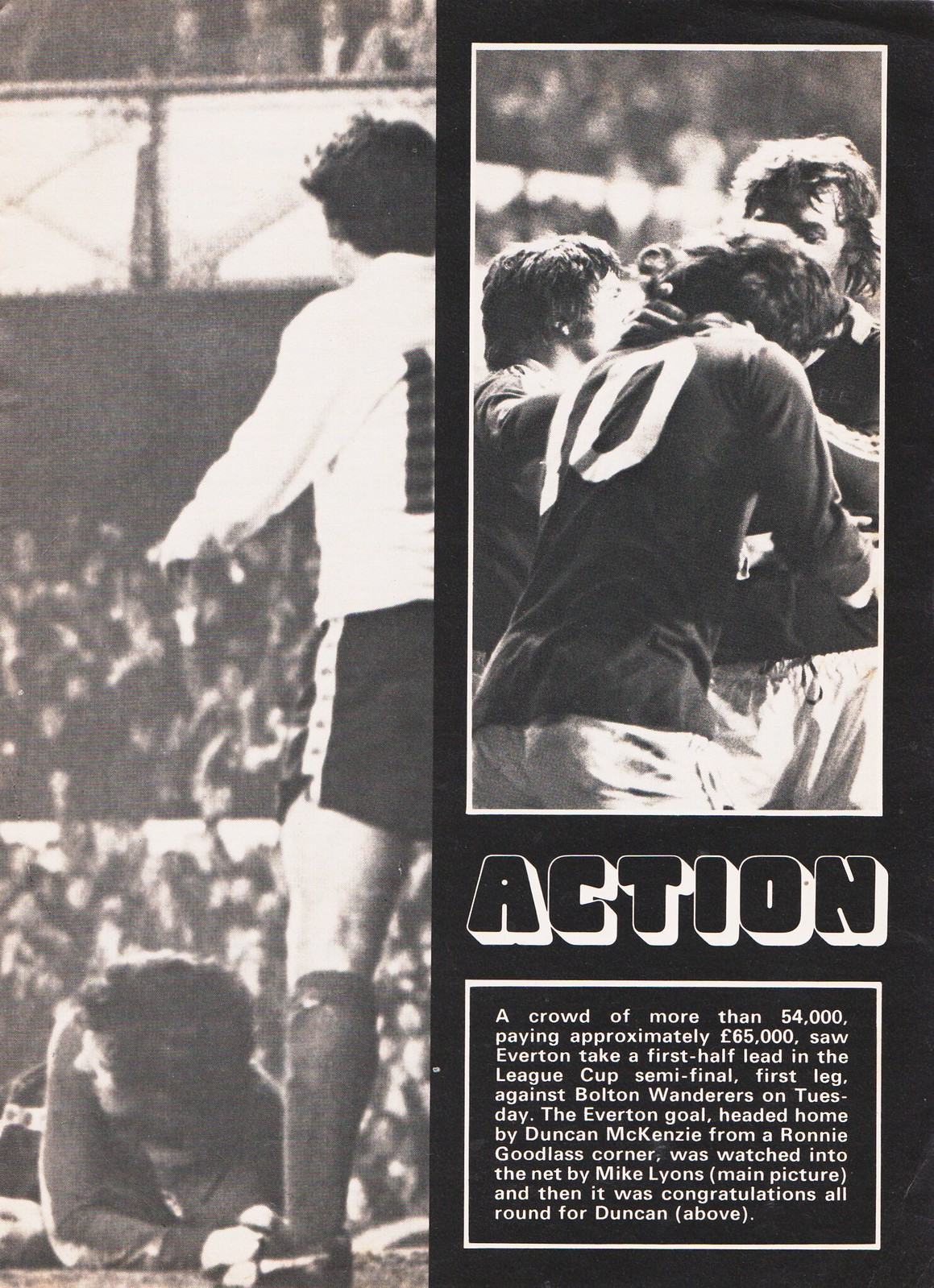The image is a black and white page from an older soccer program or magazine, featuring two distinct photographs. The main photograph, occupying the entire left side of the page, highlights a dramatic moment on the soccer field. In this picture, a soccer player wearing a white shirt and black shorts with a white stripe stands prominently, facing the left side. Nearby, another player, clad in a gray shirt, is on the ground positioned on his stomach with bent elbows, appearing as though he has just fallen. This scene is set against the backdrop of a large, three-tiered audience, their faces blurred by distance, filling the background.

The second photograph is positioned in the upper right corner of the page, showing three soccer players huddled together on a bench, captured in a moment of rest or strategizing. This image is annotated with the word "ACTION" outlined in white beneath it.

Beneath these photographs, the caption reads: "A crowd of more than 54,000, paying approximately 65,000, saw Everton take a first-half lead in the League Cup semi-final first leg against Bolton Wanderers on Tuesday. The Everton goal, headed home by Duncan McKenzie from a Ronnie Goodless corner, was watched intently by Mike Lyons, main picture. Congratulations all around for Duncan above."